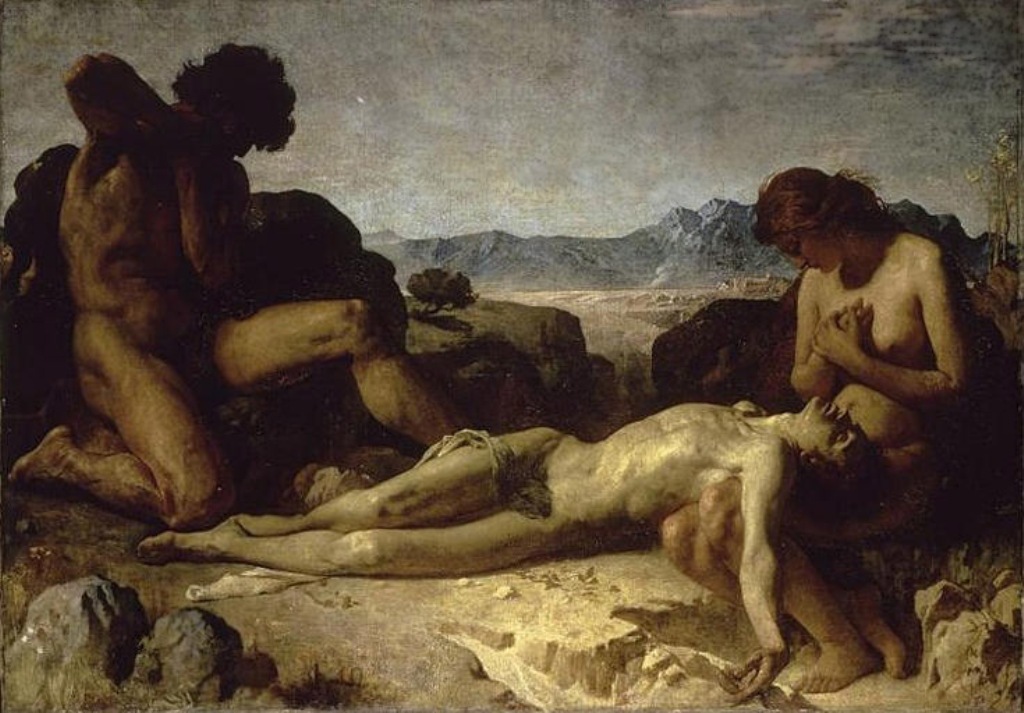The painting is a striking, photorealistic piece set in a desolate, rocky desert landscape with a distant mountain range under a dark gray sky. Central to the composition are three nude figures, their skin tones rendered in various shades of beige and pale white. On the right side of the painting, a nude woman sits, cradling the head and shoulders of an apparently deceased man in her lap, her hands clasped in a pose suggesting mourning or prayer. The man lies supine, covered only by a strategically placed loincloth, his body oriented with his feet to the left and his head to the right, gazing upwards with a lifeless expression. To the left, another nude man kneels partially in shadow, his arms folded contemplatively, possibly signifying guilt or the aftermath of a violent act. The entire scene exudes a somber, sorrowful mood, enhanced by the dull gray and beige palette. A single forlorn bush or tree in the background deepens the sense of desolation. The painting's composition and dark, evocative tone suggest it may be an allegorical or religious representation, reminiscent of the dramatic and provocative style seen in works like Goya's "Saturn Devouring His Son."